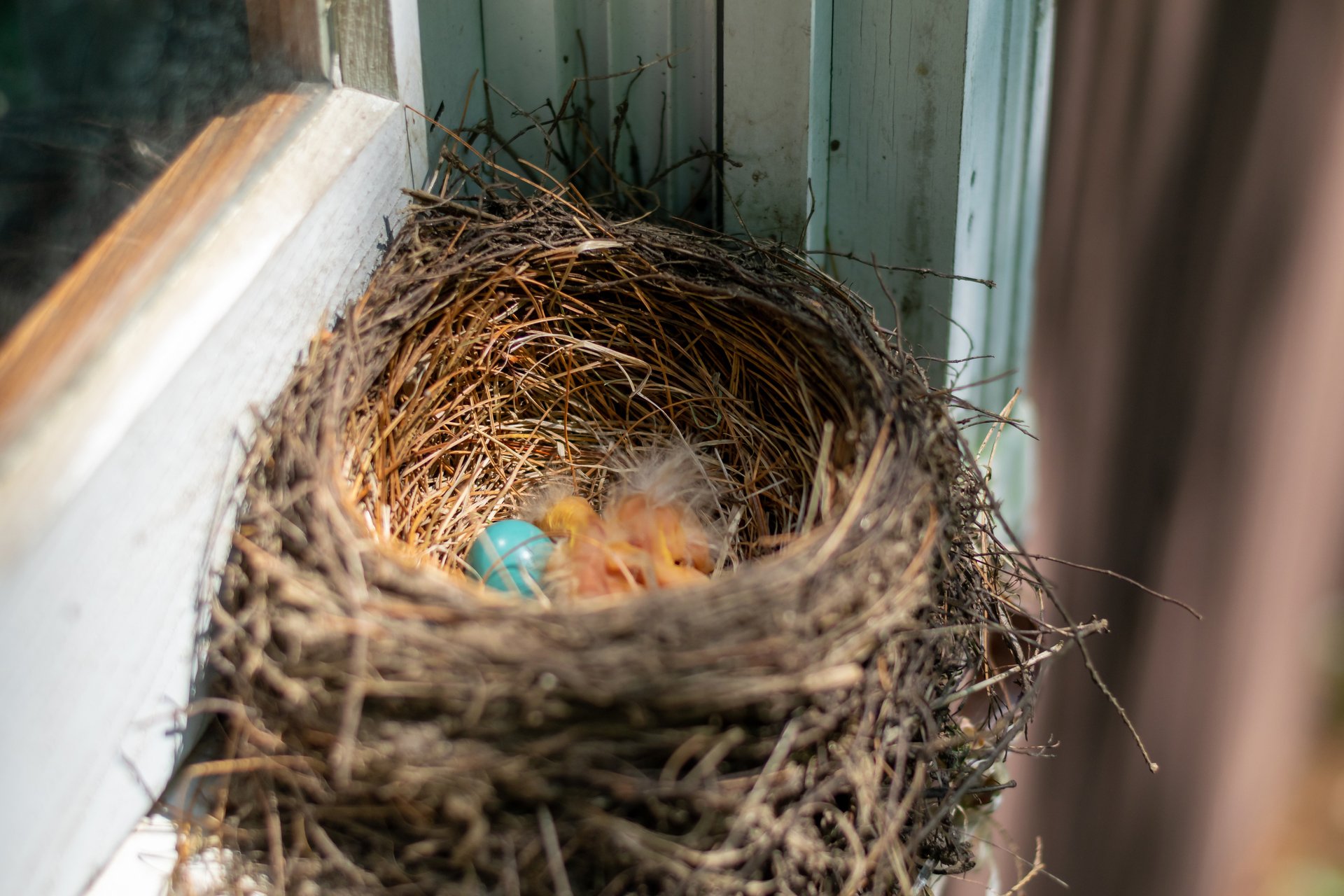The image shows a white, slightly weathered windowsill with a window on the left side. Nestled in the corner of the windowsill is a compact bird’s nest constructed intricately from pine needles, straw, and small twigs. The nest features tallish walls that somewhat obscure the interior. Inside, there are newly hatched, pink chicks with sparse white feathers, alongside a single, vivid blue egg. The scene suggests a cozy and carefully chosen spot for a bird’s home, providing a close-up look at this intimate avian setting. Out of focus, to the right, some elements remain indistinct, adding a bit of mystery to the otherwise clear depiction of the nest and its inhabitants.